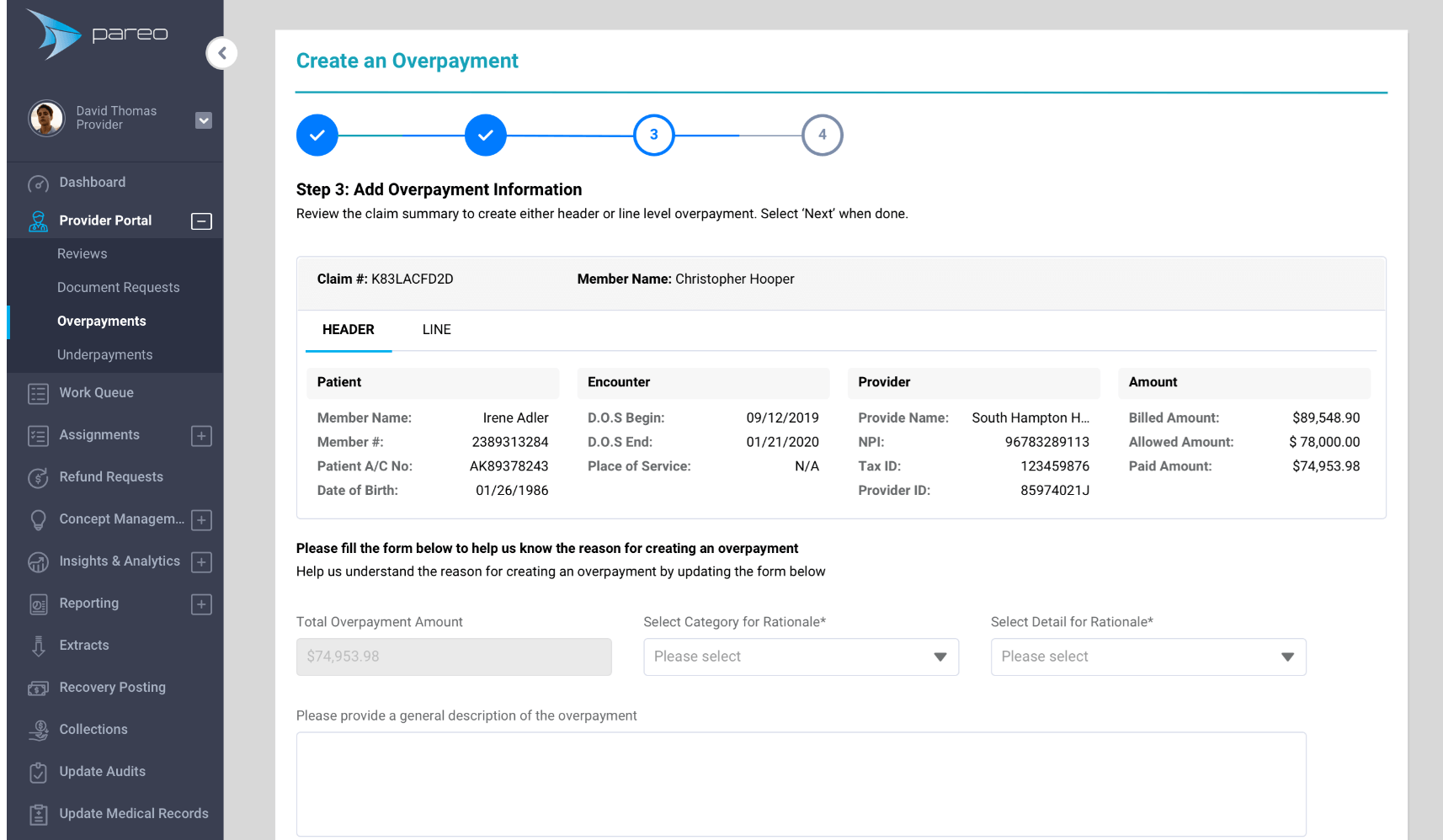The image depicts a website interface with a detailed and structured layout. In the top left-hand corner, there is a logo or text that reads "Perio." Below this, a vertical dark gray sidebar is present, featuring a small, somewhat indistinct picture of a person. Next to this image is the name "David Thomas, Provider." The sidebar lists several navigation options sequentially: "Dashboard," "Provider Portal" (highlighted), "Reviews," "Document Requests," "Overpayments," "Underpayments," "Work Key Assignments," "Refund Requests," "Concept Management," "Insights and Analytics," "Reporting," "Extracts," "Recovery Posting," "Collection," "Update Audits," and "Update Medical Records."

To the right of the sidebar, the main content area displays a white background. At the top left of this section, it has the words "Create an Overpayment." Below this, there are four instructional bubbles with two highlighted in blue and marked with white check marks, indicating completed steps. These bubbles guide the user through "Step 3: Add Overpayment Information," "Review the Claim Summary," "Create Either Header or Line Level Overpayment," and prompt the user to "Select Next When Done."

Further down, the interface lists a specific "Claim Number: K83LACFD20" followed by details such as "Member Name: Christopher Hooper." The section then bifurcates into options labeled "Header" on the left and "Line" slightly to the right, providing clear segmentation for data entry or review.